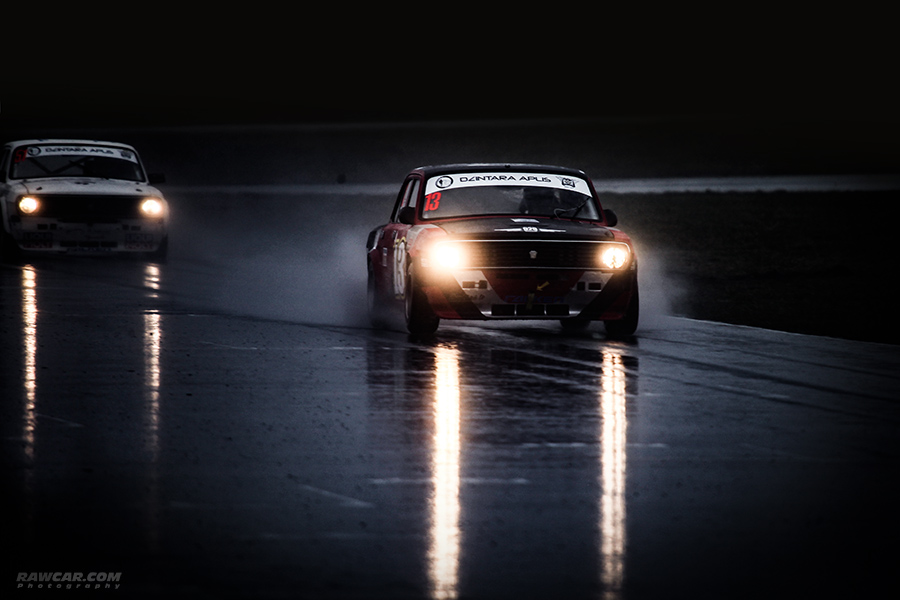The photograph portrays an intense nighttime race between two cars on a wet racetrack, their headlights piercing through the darkness with a yellow-white glow. Dominating the scene is a sleek, black car emblazoned with the number 13 on its side and windshield, leading the charge against an all-white car with a black grille, slightly obscured by motion blur. Both vehicles are captured mid-action, leaving trails of smoke and kicking up water sprays from the damp track, suggesting recent rainfall. Their powerful headlights cast reflections on the slick surface. The clarity of the image is impeccable, possibly rendered in 4K, serving to highlight details like the white bands with inscriptions across their windshields. At the bottom left corner, a watermark reads "rawcar.com - photography," identifying the specialized car photography website that captured this dramatic moment.